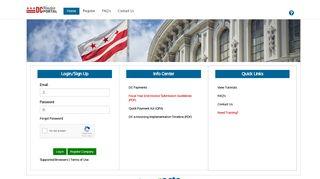In the upper left corner, a red and grey logo is prominently displayed. Below it, a rectangular blue button with white text stands out. To the right of this button, there are three additional options. In the top right corner, a blue circle contains white details within it. A stately building, crafted from grey marble, spans across a banner image, with a clear, cloud-speckled sky and a flag to its left. The flag features three evenly spaced red stars at the top, followed by alternating red and white stripes. Architectural details enhance the building's grandeur, including several palladium windows framed by decorative elements. Below these, three columns are spaced out by grey lines. Each column has a blue rectangle with white text at the top, though the text is too small to read. The first column contains two rectangular boxes, a grey box, and two green rectangular buttons at the bottom.